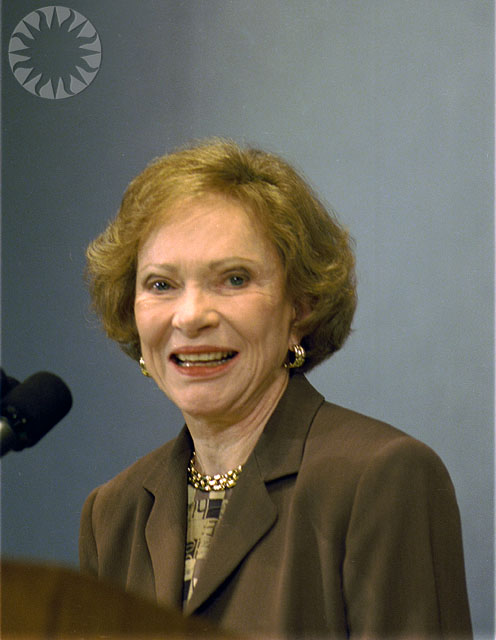This detailed photograph captures an elderly woman, potentially a former First Lady, dressed in business attire that includes a medium brown suit jacket and a checkered blouse in shades of cream, brown, and black. The top half of her body and head are in focus, revealing her short, golden-brown hair with a hint of red and a warm smile adorned with coral-colored lipstick. She accessorizes with gold hoop earrings and a thick gold necklace. The woman is standing in front of a microphone, which peeks into the frame from the left side, contributing to the professional atmosphere suggested by the potential presence of a podium, partly visible in the foreground. A solid light gray wall forms the backdrop, with subtle shading differences due to lighting. In the top left corner of the image, a white circular watermark featuring a cut-out sunburst design is visible, adding a distinct but unobtrusive mark to the photograph.